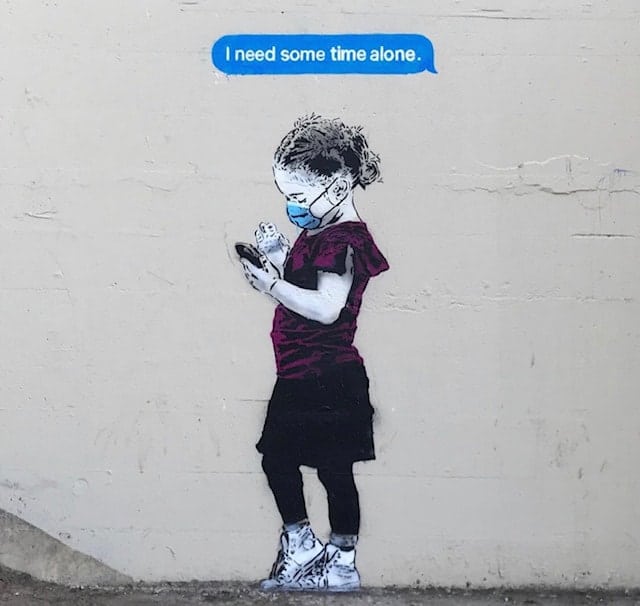The artwork, painted on the side of an older building with a weathered white exterior wall, portrays a young girl looking down at a smartphone she holds in her left hand while interacting with it using her right hand. The girl, who might be in her early childhood years, has short, curly dark hair tied back and wears a blue surgical mask. Her attire includes a purple blouse with slit cap sleeves, a black dress over black leggings, and white high-top basketball sneakers. Above her head, within a blue thought bubble written in white letters, are the words, "I need some time alone." The textured wall, marked with some filled-in cracks, emphasizes the mural's setting in a period reflective of the COVID-19 pandemic, likely around its early days.